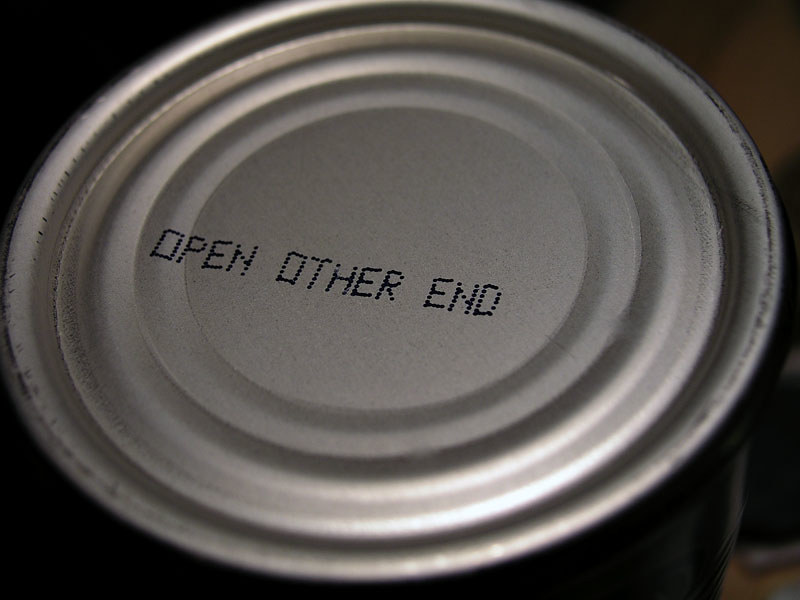This close-up photograph captures the bottom of a bright, silver aluminum can. The lid is marked by several concentric circles and grooves that radiate outward from the center, adding to its intricate texture. Written in the center in typeset, black, dot-matrix style letters are the words "OPEN OTHER END." The can’s surface has a few scratch marks and stains along the outer edge, indicating wear. The background features indistinct blobs of black and orange, contrasting the shiny, metallic appearance of the can.